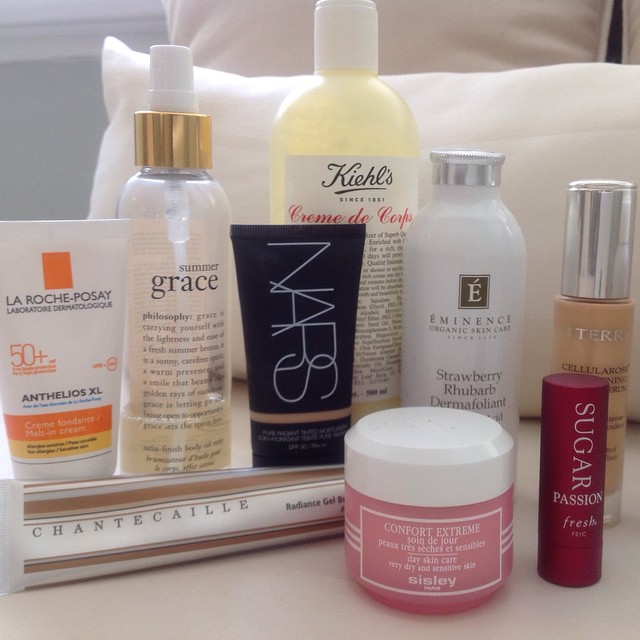The photograph showcases an array of personal care products meticulously arranged on a pristine white surface. Against the backdrop of a white wall and a small white and tan pillow, the assortment of products includes:

1. A tan and white packaged item with black font, which reads "CHANTECAILLE".
2. A La Roche-Posay tube, predominantly white with orange and yellow accents and black font.
3. A clear bottle with a white and gold cap, labeled "Summer Grace" followed by black text beneath it.
4. A sleek black tube inscribed with white font, identified as a product from NARS.
5. A bottle from Kiehl's, featuring a white label with black text and a matching white lid.
6. A white bottle adorned with a silver cap, stating "Eminence" in brown font and "Strawberry Rhubarb Dermafoliant" in black.
7. A pink jar capped with white, displaying "Comfort Extreme".
8. A burgundy tube with white lettering, marked as "Sugar Passion Fresh", likely a lip product.
9. Finally, a tan product with a silver lid, detailed with silver and black font, positioned slightly behind the other items.

The careful arrangement highlights the diversity and elegance of each personal care product, creating a visually appealing and detailed display.